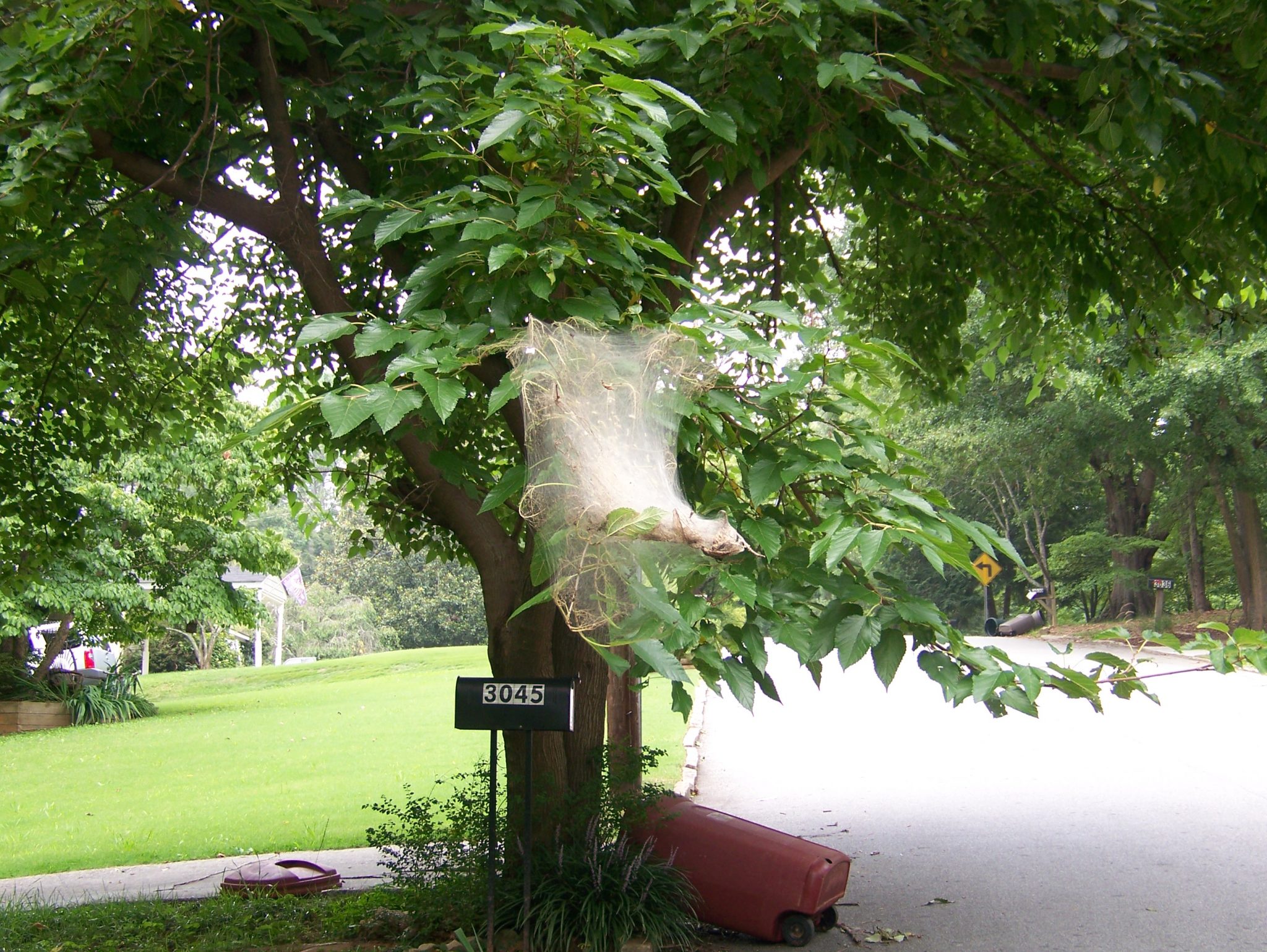The image depicts a tree in someone's backyard, prominently covered in a large, white web capsule, likely formed by caterpillars such as tank caterpillars. The entire branch is ensnared in webbing and silk, with a few caterpillars visible at the top, possibly feeding on the leaves. This tree is centrally located and flanked by lush green leaves, indicating either late spring or summertime. Below the tree, a black mailbox marked with the number 3045 stands out, with white stickers displaying the numbers. Next to it lies a knocked-over magenta dumpster, with its lid discernible in the driveway close by. In the background, additional details include a white car with a red taillight to the left and a yellow road sign with a left turn arrow further down the road. Additionally, across the street, there's a smaller mailbox from another property. The scene is framed by more mature trees with large brown trunks, enhancing the contrast with the vibrant greenery and the striking, web-covered tree.